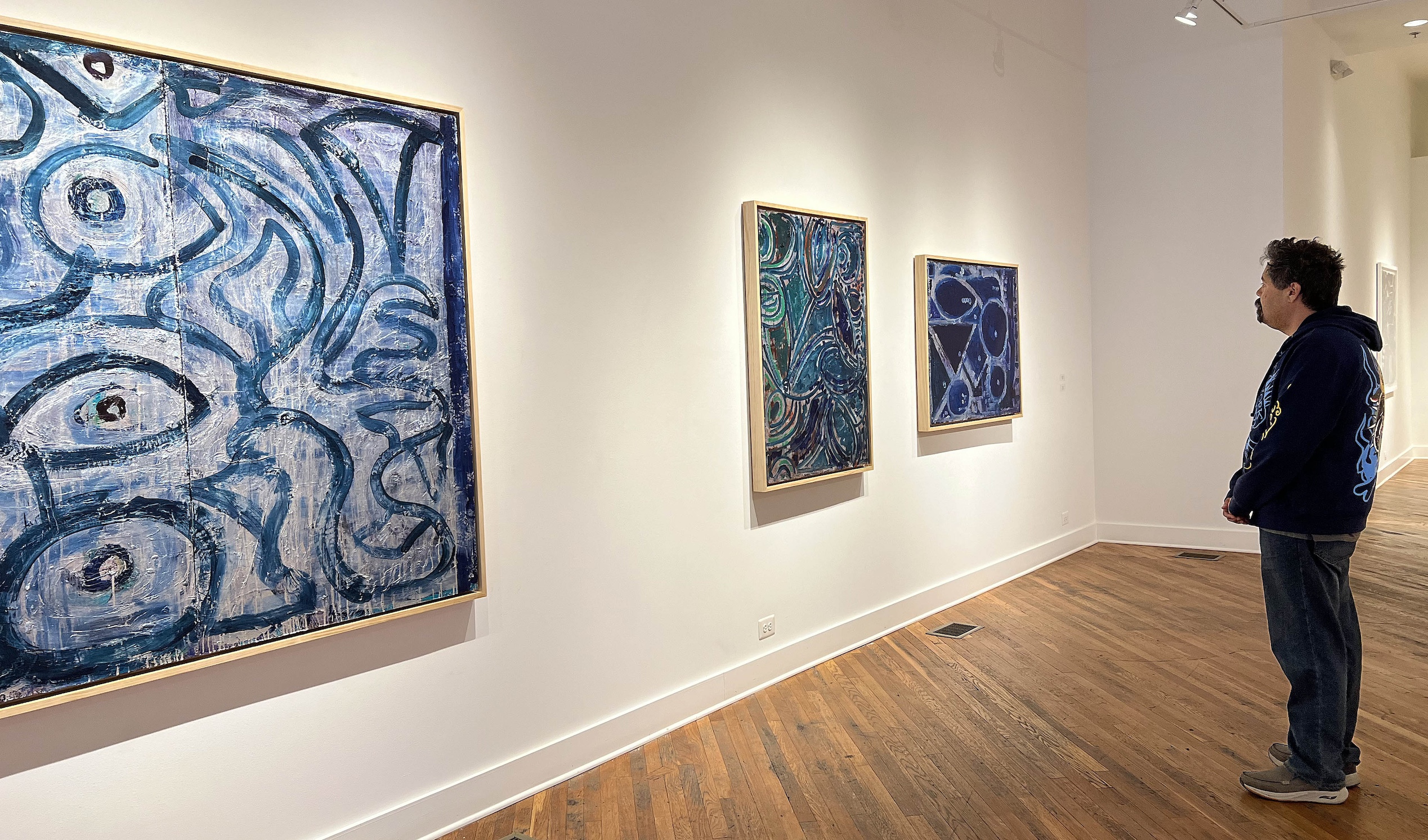In this horizontal rectangular image taken in an art museum, we see a man standing opposite a wall adorned with three paintings by the same artist, all utilizing varying shades of blue. The gallery's floor is polished brown wood, while the walls are pristine white, casting shadows under the gallery lights. The man, with dark hair, a beard, and a mustache, is dressed in a black hoodie featuring blue designs, blue jeans, and grey sneakers with white soles. His hands are in his pockets as he contemplates the artwork. The paintings, each set in gold metal frames, showcase abstract designs; the nearest one features circles, while the others, despite sharing the same blue tones, exhibit distinctly different patterns. The middle painting is notably colorful, incorporating swirls and dots, whereas the final, smallest piece, presents a simpler composition of just a few shapes. The room also includes details like a wall socket, floor vents, and ceiling lights, contributing to the gallery ambiance.